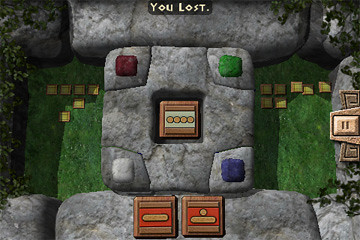This is a screenshot from a video game featuring a centered message in white font that reads "You Lost." The image is horizontally aligned with large gray stone formations placed along the top and bottom edges. In the middle, there's a large square made of the same gray stone material, segmented into smaller regions marked by colored squares at each corner—reddish-brown in the upper left, green in the upper right, light blue in the lower right, and whitish-gray in the lower left. At the very center of this square is a tan rock with four yellow dots arranged horizontally. The background behind these stones appears to be green grass, with some small green squares dotted across it. At the bottom of the image, there are two glyphs, each housed in wooden-framed squares with two brown bars over a red field, featuring either a line or a line and a dot.